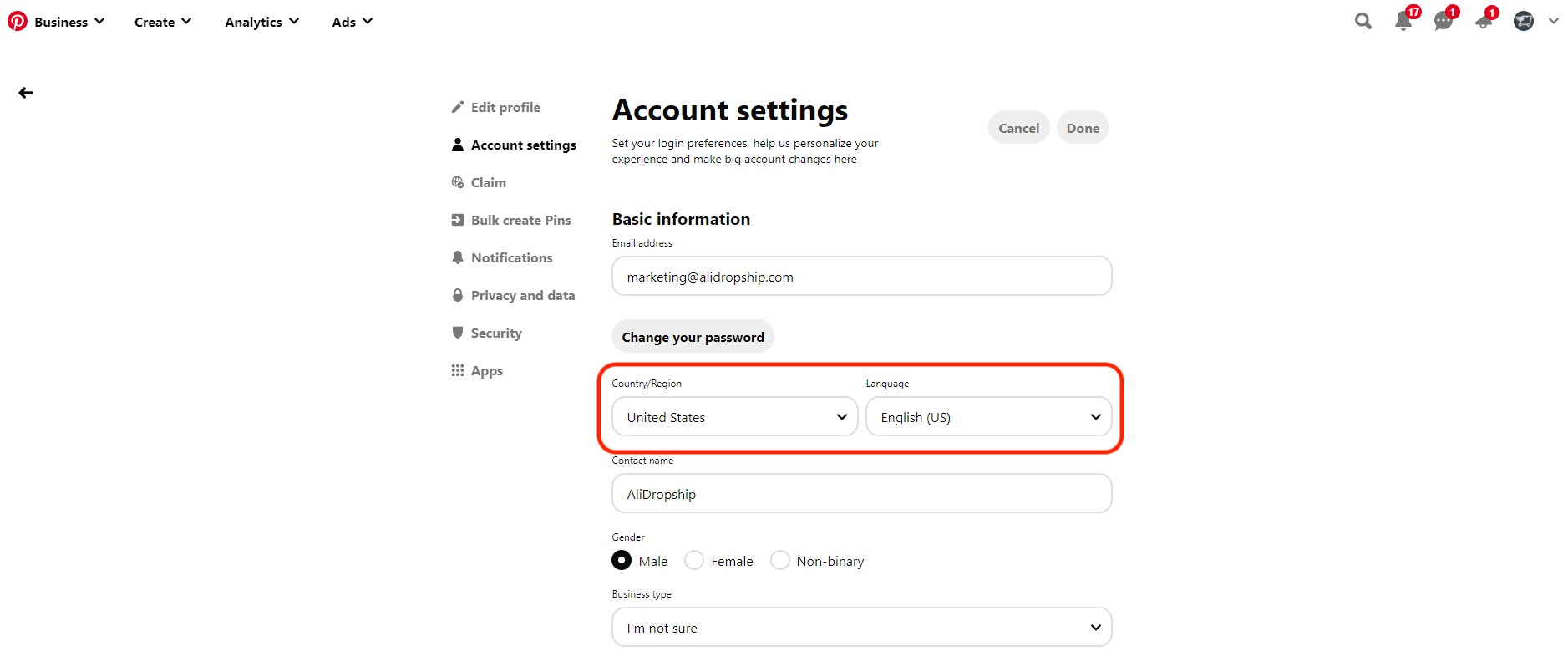This is a detailed description of a website's account settings page:

At the top-left corner of the website, there is a prominent white "P" encapsulated within a pink circle. This is followed by large text categories labeled "Business," "Create," "Analytics," and "Ads."

Centrally located under the main navigation, the header "Account Settings" is displayed in bold, dark black text. To the left of this header, there is a vertical menu with several options:
1. "Edit Profile"
2. "Account Settings" – a brief description below it reads, "Set your login preferences, help us personalize your experience, and make big account changes here."
3. "Claim"
4. "Bulk Create Pins"
5. "Basic Information" – with further sub-options like:
   - "Email Address" accompanied by an input box.
   - "Security" – with a "Change your password" box under it.
   - "Apps"

In the central highlighted section circled in red, users can configure the following settings:
- "Country/Region" with a dropdown menu currently set to "United States."
- "Language" with another dropdown menu set to "English (US)."
- "Contact Name" displaying "ALI DROP SHIP."
- "Gender" options including "Male," "Female," and "Non-binary."
- "Business Type" with a dropdown menu currently displaying "I'm not sure," allowing users to select various business types.

This detailed layout ensures users can efficiently navigate and customize their account settings.